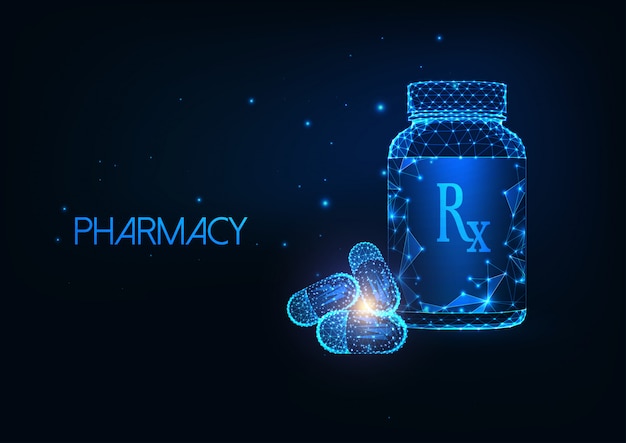This detailed blue-toned digital artwork features a dark blue background adorned with the word "PHARMACY" in all caps on the left side, with the unique detail of the A's being slanted to the right. Surrounding the word are light blue, glowing pinpricks that resemble stars in a night sky, lending a constellation-like appearance. On the right half of the image lies a futuristic, geometric line art depiction of a pill bottle with a screw cap, marked with an opaque blue label reading "RX." In close proximity to this bottle, three large gel capsule pills, half light blue and half dark blue, are meticulously stacked in a pyramid shape, with a glowing white spot of light emitting from their center. The entire composition exudes a high-definition, neon blue aesthetic, as if formed by digital stars or points, reminiscent of a 3D model in the making.